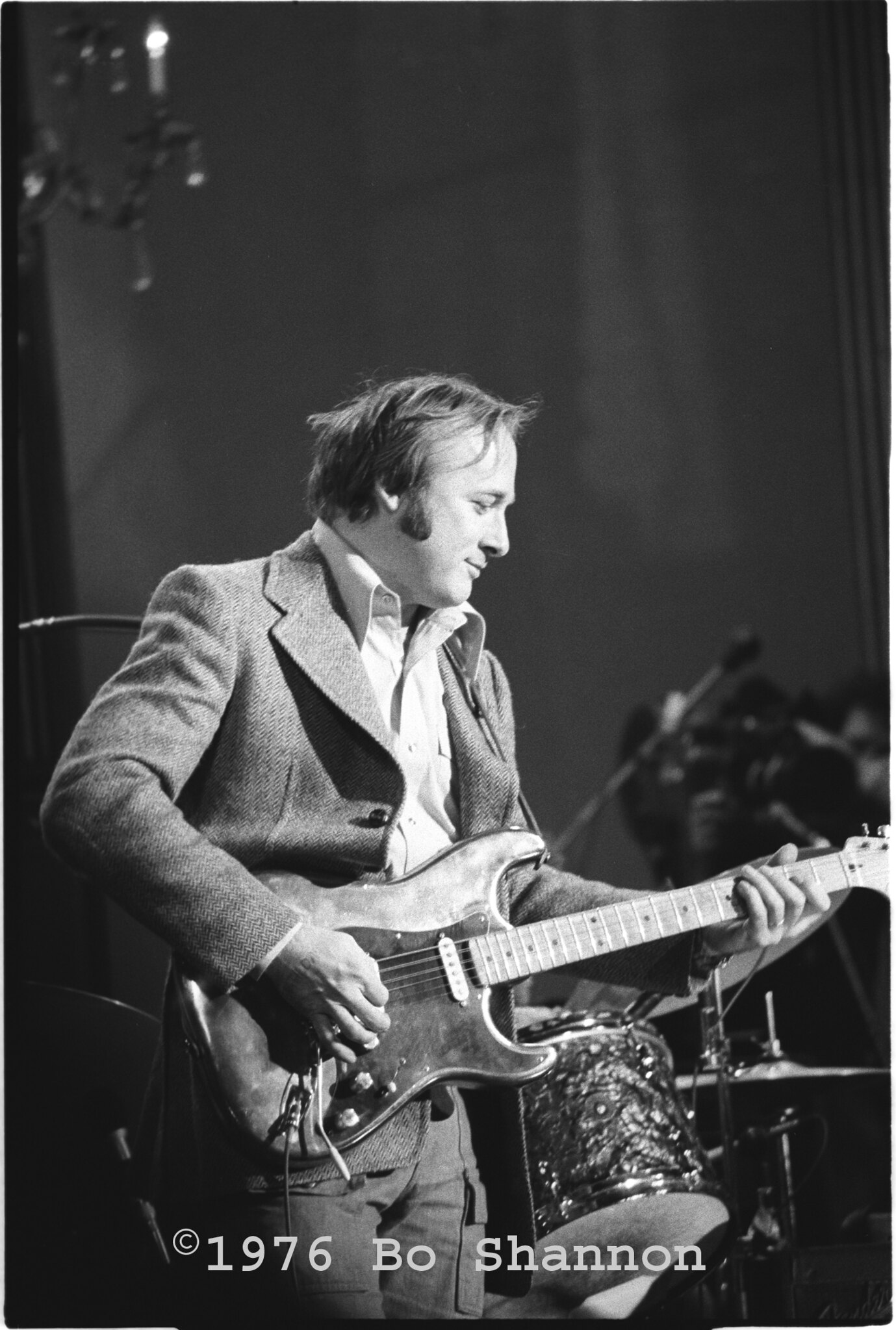In this evocative black and white photograph dated 1976, captured and possibly taken by Bo Shannon, a man identified by some as Van Morrison takes center stage. This musician, appearing to be in his early 30s, stands poised with an electric guitar in hand, showcasing a white pickup in the front. He is dressed smartly in an unbuttoned tweed sport coat over a white collared shirt devoid of a tie, revealing a sense of casual refinement. His balding forehead is complemented by long hair that covers his ears and sideburns that extend just past them. Behind him sits an unattended drum set, a testament to the venue’s readiness for an ensemble. The backdrop is adorned with flowing white curtains, and a chandelier hangs above, suggesting not just any stage, but one of elegance. There seems to be an audience member barely visible at the bottom right corner of the image, hinting at a live performance. The photograph encapsulates the essence of a moment in musical history.